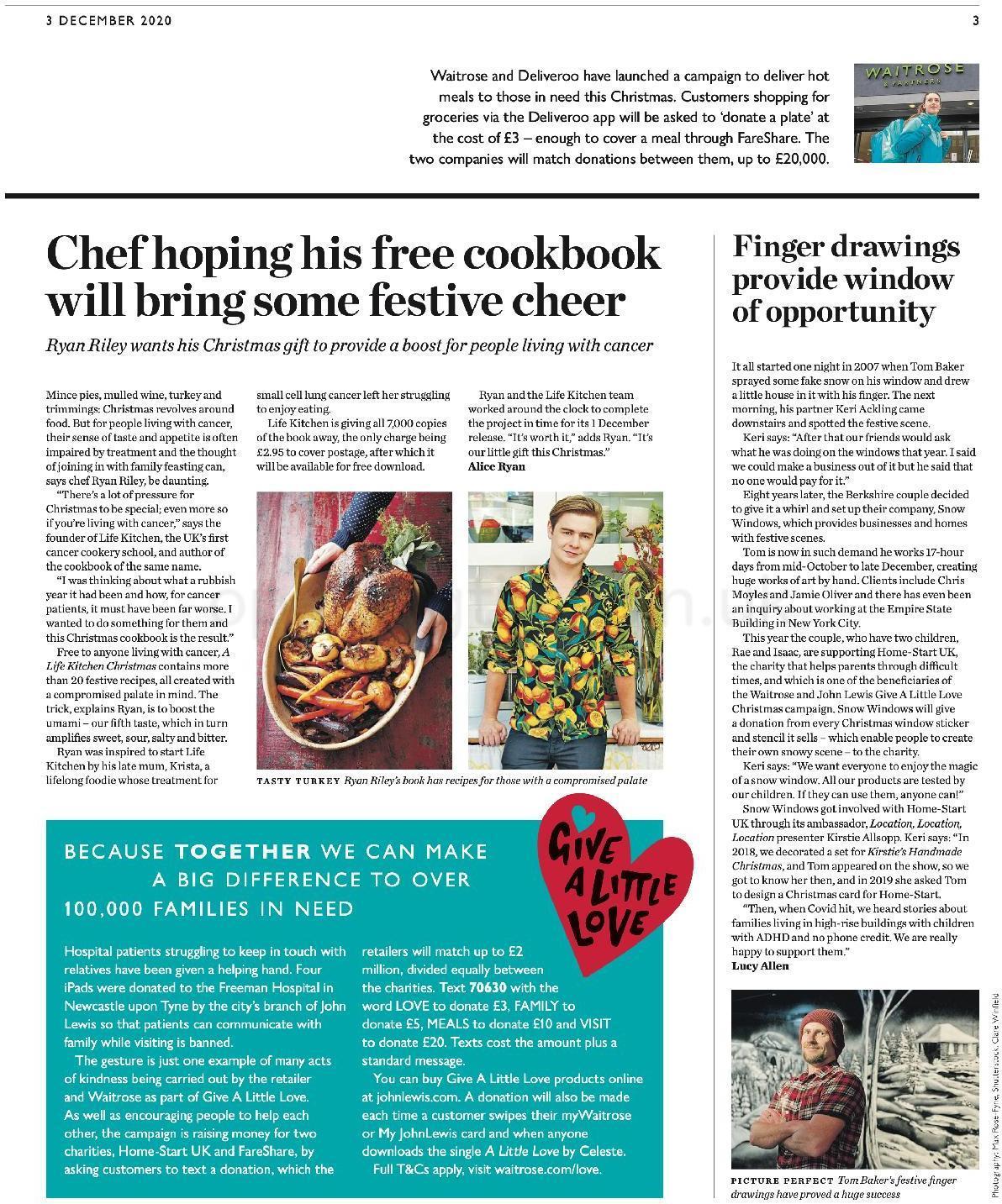This detailed and polished caption provides a thorough description of the newspaper screenshot:

The image is a screenshot of what appears to be the front page of a newspaper dated December 3, 2020. In the upper left corner, the date is prominently displayed. In the top right corner, there is a small photograph of a woman wearing a blue jacket and carrying a backpack. To the left of her image, some text is present.

Centrally positioned is a large headline accompanied by an article titled "Chef Hoping His Free Cookbook Will Bring Some Festive Cheer." The article details how Ryan Riley, the chef, aims to uplift the spirits of individuals living with cancer through his Christmas gift.

In the center of the page, there's a vivid photograph of a ceramic dish filled with a festive meal, including turkey, carrots, and potatoes. To the right of this image, another picture features Ryan Riley. He is a young white man dressed in a green shirt with yellow food prints and wearing jeans.

Below this central area, a blue box contains additional information. In the upper right corner of this section, a small red heart icon accompanied by the text "Give a Little Love" is noticeable.

On the right side of the page, a narrow and lengthy article titled "Finger Drawings Provide Window of Opportunity" is present. Towards the bottom right, there's a photograph of the artist—a white man in a hat and a red plaid shirt. A drawing of a house and some land can be seen in the background behind him.